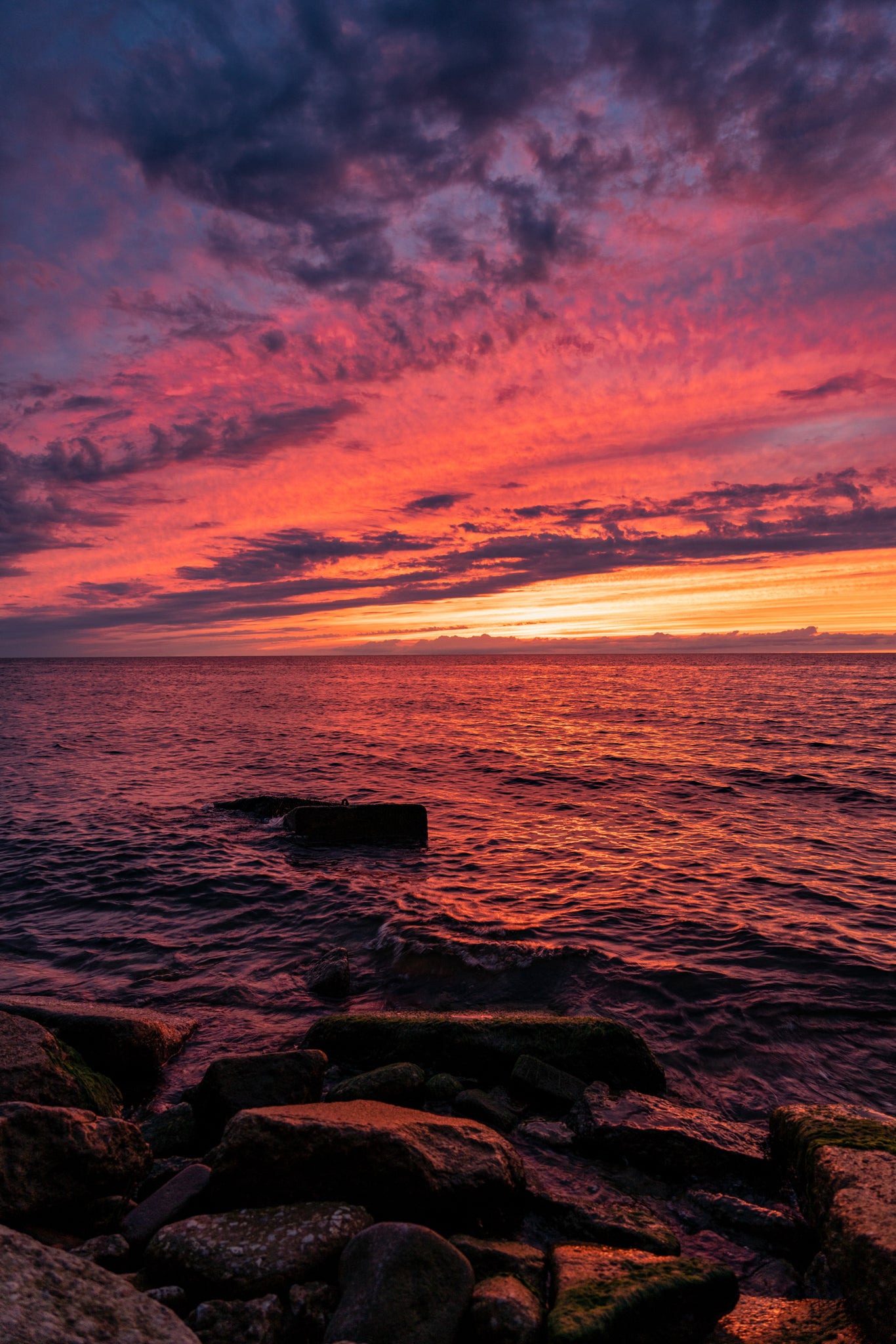This is a realistic photograph of a tranquil beach scene at dusk, vertically oriented and taken outside during the day. In the foreground, there are numerous large, square and oblong rocks scattered near the water's edge, about 15 in total with one rock protruding slightly further into the water. The ocean, calm with slight ripples, extends across the bottom half of the image, reflecting the stunning colors of the sky above. The water captures hues of orange, pink, and purple from the sky, devoid of visible waves but rich in texture.

The horizon divides the photograph, with the top half dominated by a dramatic, cloud-laden sky. Right above the horizon, the sun, visible through a cluster of clouds, radiates the brightest and most vivid yellow, transitioning to orange, red, and blue as it ascends. The sky culminates in deep purples at the top, fading into darker shades away from the light. The clouds present a varied texture, showing horizontal striations closer to the horizon and becoming puffier towards the top of the image. This photorealistic image captures the serene beauty of the sunset, with its vivid array of colors and the calming interplay of the sea and sky. There are no text elements in the image, allowing the natural beauty to speak for itself.